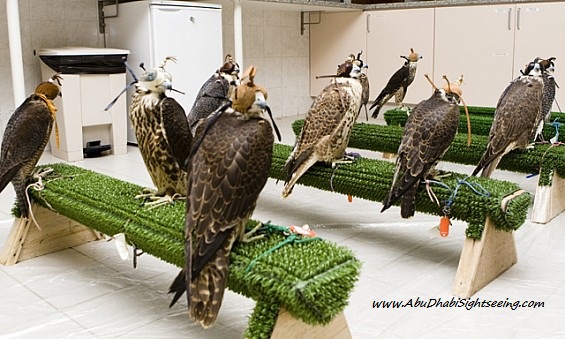The image features a group of 9 falcons inside a building, all wearing colorful hooded masks used for training by falconers. The falcons are perched in rows of three on four benches, each covered in artificial green turf. The background displays an off-white wall with cupboards featuring silver handles, a white refrigerator, and a large off-white trash can with a black foot pedal. The floor is primarily off-white with some brown. This organized layout suggests a veterinarian’s office or a facility dedicated to falconry. On the bottom right corner of the image, the text “www.abudabisightseeing.com” indicates it might be an advertisement related to sightseeing or falconry activities.